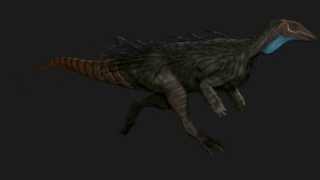The image depicts a small, intricately detailed dinosaur running to the right, set against a nearly black background. The dinosaur resembles a velociraptor with a unique mix of features: it has long, powerful legs akin to a bird's, and much shorter arms. Its body, which appears to be covered in a mix of tan fur and dark feathers, seems slightly balding in places. The dinosaur sports a white throat and a head that combines the traits of a plant eater and an anteater, with a long snout and beak-like nose. The tail is notably long and ridged, resembling that of an armadillo with vertical black rings, while its back is lined with spikes. The overall color of the dinosaur is dark, with varying shades of dark green, brown, and hints of orange.